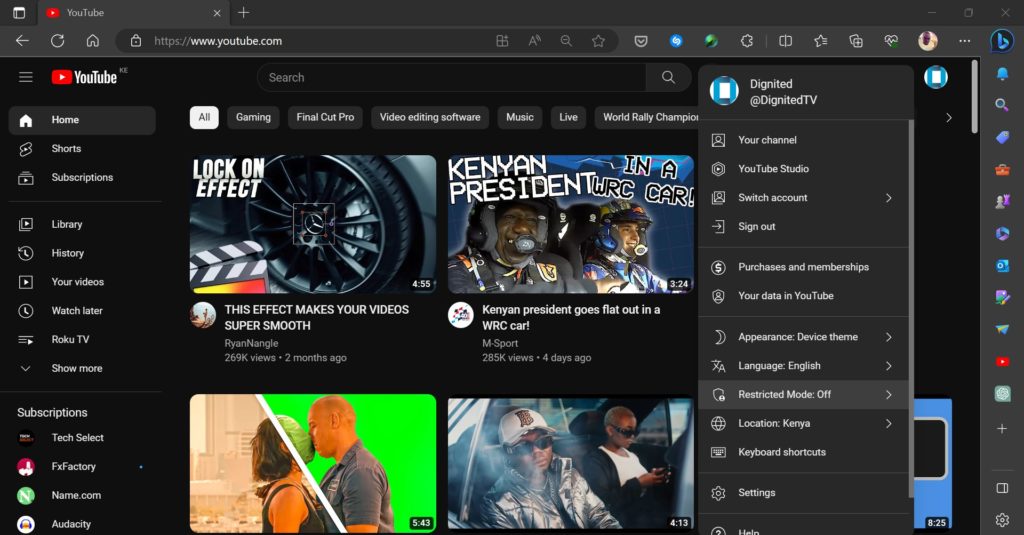**Caption:**

This image showcases the YouTube website interface on a black background with white text. At the top, the browser's search bar is visible with "YouTube" typed in. Just below the search bar on the top left, the YouTube logo is prominently displayed. On the far left side of the page, there is a vertical sidebar featuring a menu with various selectable buttons: Home, Shorts, Subscriptions, Library, History, Your Videos, Watch Later, and Roku TV. There's an additional option labeled "Show More" which reveals a drop-down box.

Under the Subscriptions section, there are text entries displaying "Text," "Select," "FX Factory," "Name.com," and "Audacity." Centrally located below the search bar, another set of buttons categorizes content into: All, Gaming, Final Cut Pro, Video, Video Editing Software, Music, Live, and World Rally Champion.

The main content area beneath these buttons displays four video thumbnails. The first video is titled "The Lock-On Effect," the second is "Kenyan President," the third thumbnail features two people kissing with one half of the box in green, and the fourth video depicts two individuals sitting in the backseat of a car, with one looking at a cellphone and the other appearing to blow smoke.